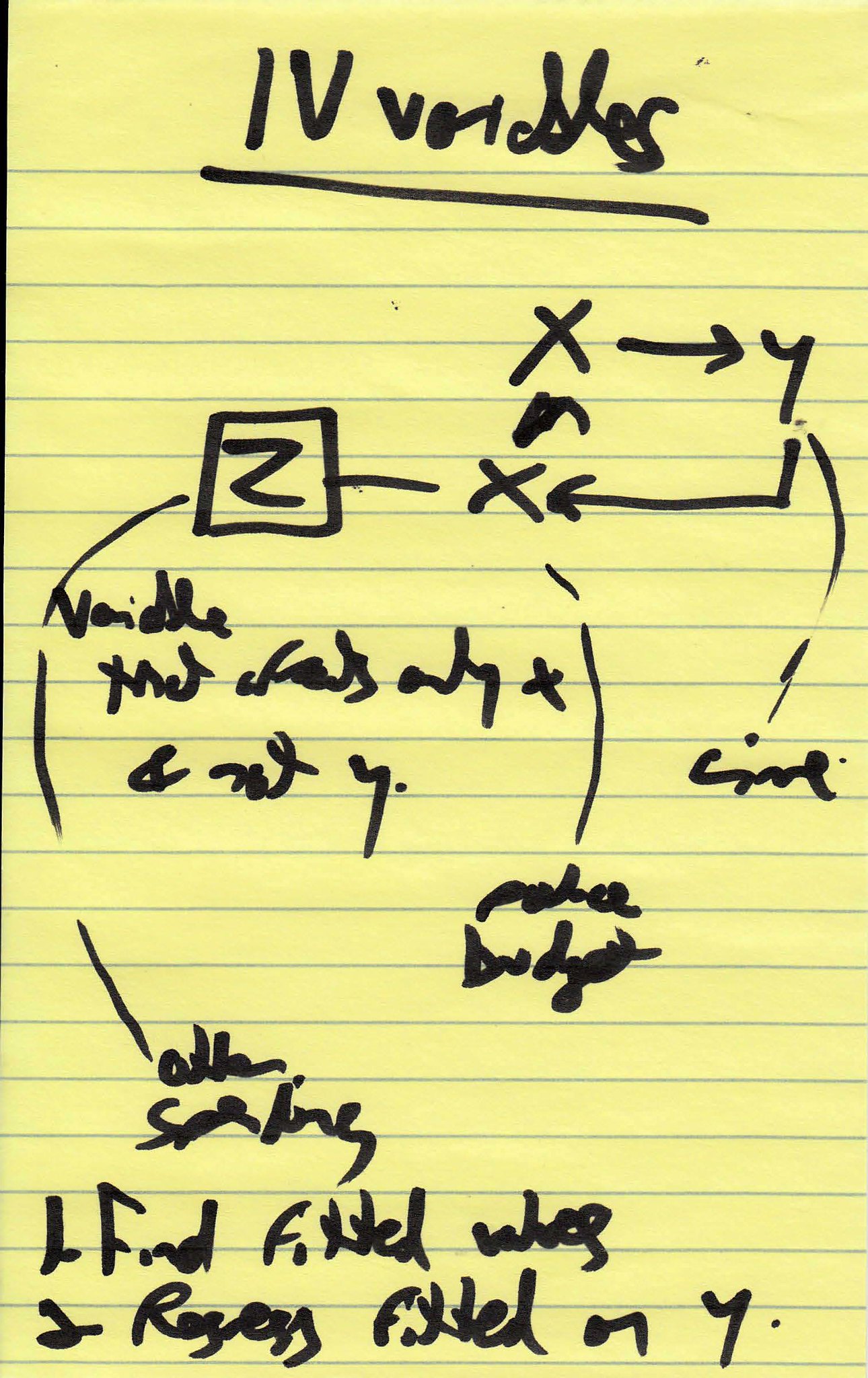Close-up of math notes written in black magic marker on yellow, lined notebook paper. The notes feature the heading "Roman Numeral IV - Variables" and include various algebraic expressions, diagrams, and equations. The handwriting is quite sloppy and difficult to decipher, adding to the challenge of interpreting the mathematical concepts presented. The yellow notepad with blue lines is typical of a standard legal pad, and the entire scene suggests the hurried, impromptu nature of someone's algebra study session.